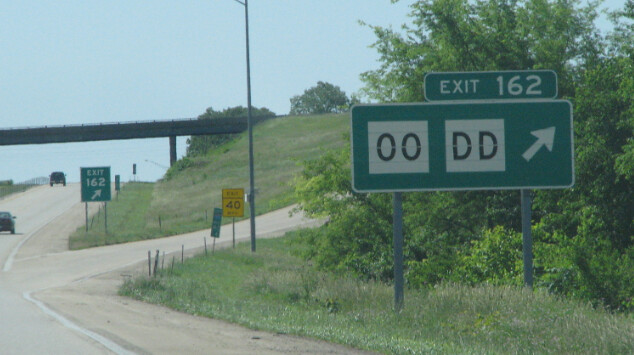The image showcases a highway curving slightly to the right, indicating the photographer is likely in a moving car. There are two vehicles ahead: a black sedan and a black truck, both driving on the gray-colored road. The right side of the highway features green grass and brush leading up to an exit marked as 162, with a prominent green rectangular sign displaying "EXIT 162" with an arrow directing to the right. There is also a smaller green sign and a yellow rectangle indicating a speed limit of 40 miles per hour, although parts of the text might be partially obscured. A gray bridge spans across the highway, supported by a visible leg, and no vehicles are present on it. Beyond the highway and around the exit path is a large hill with green and some patches of dead grass, topped with green trees. The sky is clear and blue, providing a serene background to the scene.